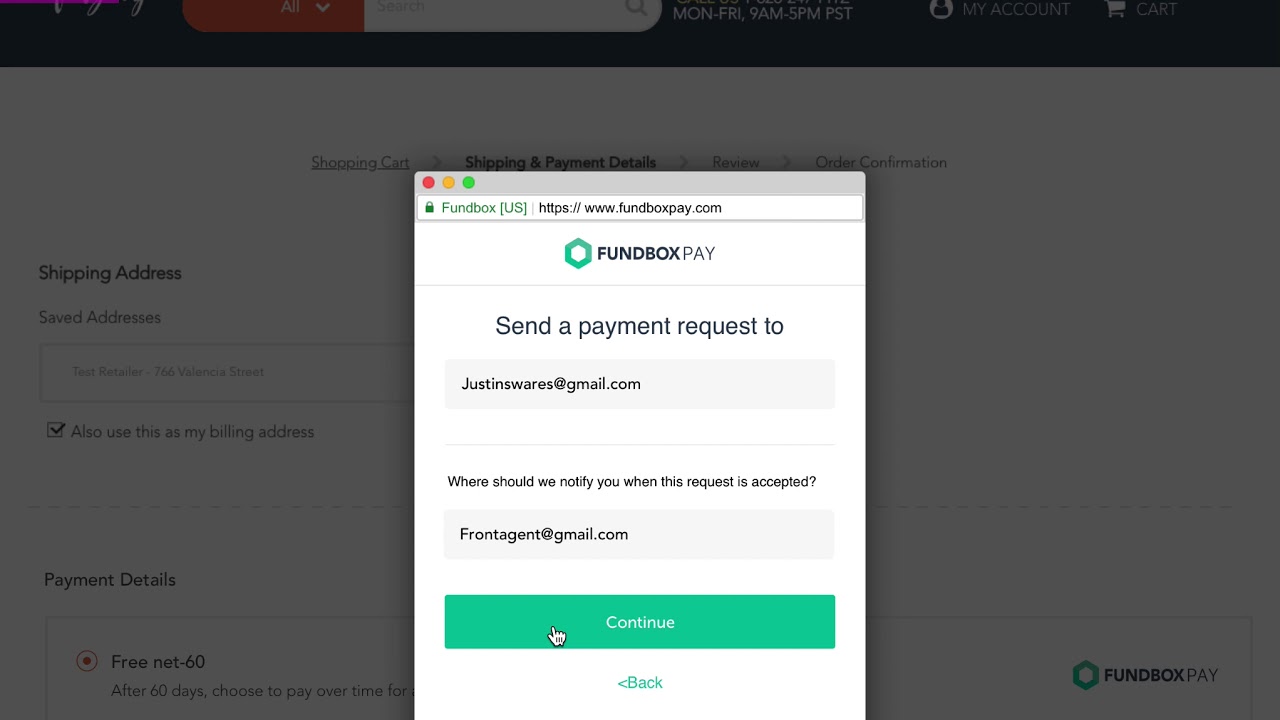This image is a screenshot from a website, partially obscured by a pop-up box in the center. The webpage itself appears grayed out, but certain elements are still discernible. The background seems to be light-colored, with a header at the top that is darker in color. Though not clearly visible, the company's logo appears in the bottom right corner, indicating this is FundBoxPay. The name "FundBoxPay" is written as one word, with "FundBox" in bold font and "Pay" in regular font. Adjacent to the text is a pentagon shape outlined in green, with a white interior.

In the pop-up box positioned centrally on the screen, the same FundBoxPay logo is prominently displayed. The pop-up features a top border in a light gray color. On the left side of this border, there are three small dots: one red, one yellow, and one green. To the right of these dots, the web address FundBoxPay.com is displayed.

Below the logo within the pop-up, the text reads: "Send a payment request to" followed by the email address "justinswares@gmail.com". Further down, a question is posed: "Where should we notify you when this request is accepted?" Directly beneath this question is another email address: "frontagent@gmail.com". 

At the bottom of the pop-up box, there is a green rectangular button with the word "Continue" written in white. Beneath this button, against the white background of the pop-up, the word "Back" is written in green, accompanied by a left-pointing arrow.